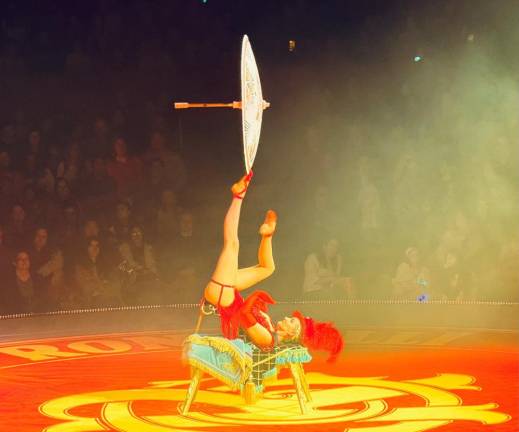This image captures a mesmerizing scene from a circus show, potentially from Cirque du Soleil, featuring a stunning circus performer in mid-act. She is elegantly laying on a bench at the center of a circus tent, surrounded by an intrigued audience. Despite the misty and blurry background, the spectators appear slightly impressed as they gaze upon her display.

The performer is adorned in an all-red outfit, which includes a unisuit or bunny suit that exposes her legs, red gloves that cover her arms, and a striking red hat adorned with a feathered boa. Her feet are accentuated by red high heels or slippers. One of her legs is lifted high into the air with an elegant arch, and at the tip of her outstretched foot, she is skillfully balancing an open parasol. Her right leg is bent gracefully at an angle, adding to the poise and complexity of her performance. The floor beneath her is a deep red with intricate yellow designs, complementing her vibrant attire.

With her eyes fixed upwards and a serene expression on her face, she captivates the audience, all of whom are visible through the dim haze, contributing to the enchanting and almost surreal atmosphere of the scene.